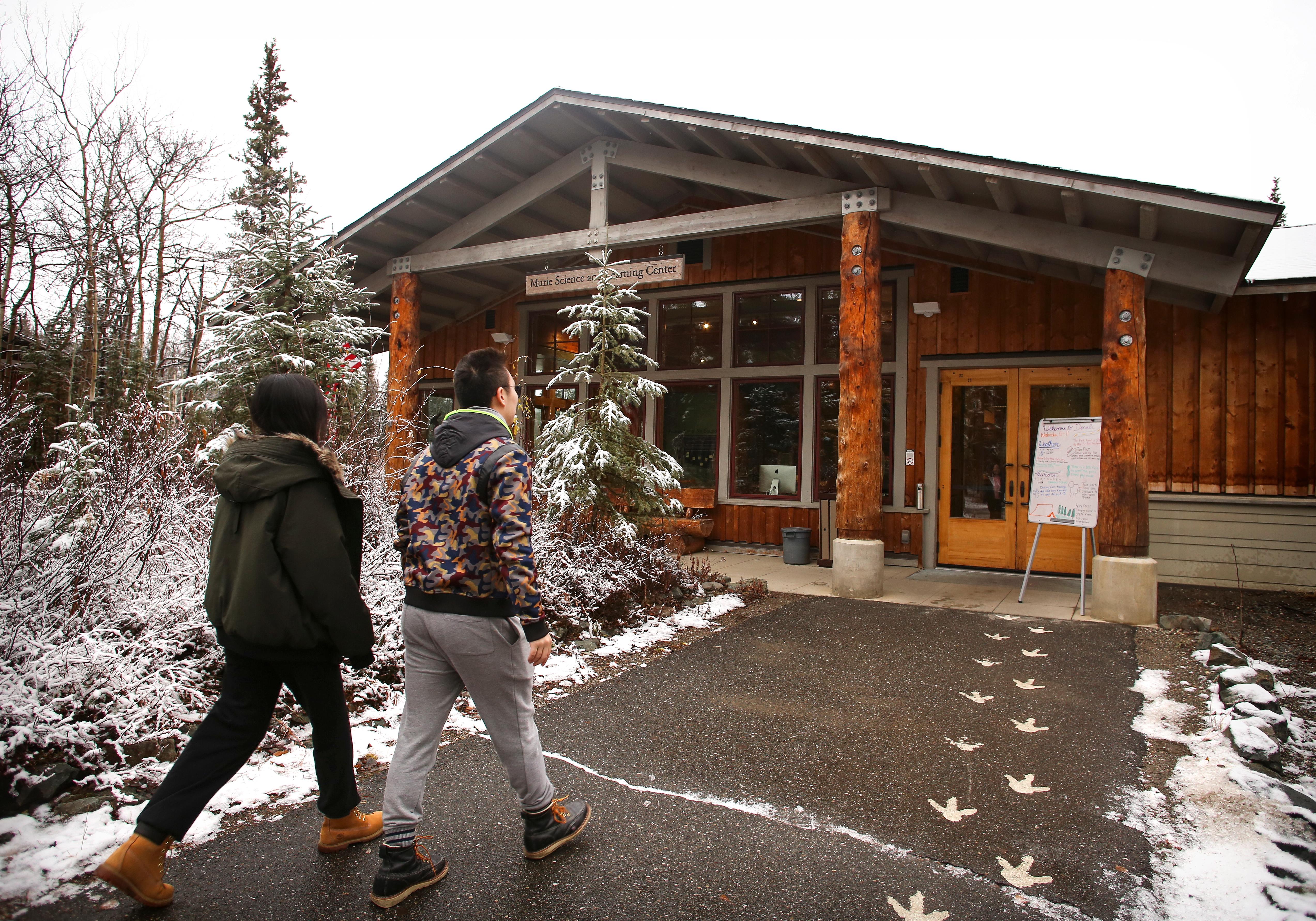The photograph captures a picturesque winter scene featuring two people walking towards a rustic wooden cabin, identified by a sign as the "Murie Science and Learning Center." The cabin resembles a traditional log cabin with a triangular roof, constructed from wooden beams and logs, possibly featuring a corrugated iron roof. The building is set in a serene, snow-covered landscape with trees dusted in snow flanking both sides. The couple, a man and a woman, are dressed warmly in winter attire, including thick jackets, coats, and boots. The man wears a camouflage hooded jacket, grey tracksuit bottoms, and black boots with orange laces, while the woman sports a green parka with a fur trim, dark trousers, and rust-colored boots. They walk on a wide, paved pathway leading up to the entrance, beside which stands a whiteboard on an easel with indistinguishable writing. The presence of multiple windows hints at a cozy interior meant for learning and community activities. The bright, snowy day gives the scene a tranquil, inviting atmosphere, with the white sky suggesting it is daytime. The overall setting suggests a remote, peaceful locale, possibly within a forest or a park, designed for educational purposes amid nature.